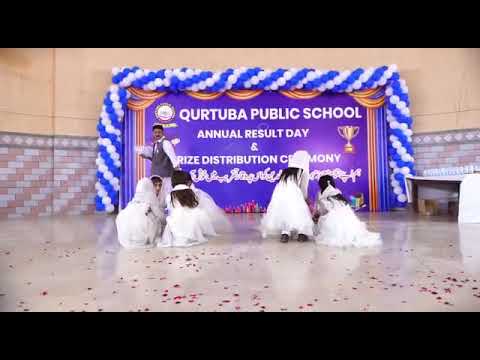In this image, several young children dressed in fluffy white dresses and headgear are positioned in two small groups, centered near the bottom of the image. To the right of one group stands an older man dressed in a gray vest over a white shirt, looking down at the children. The scene is set on a polished, shiny floor that has some scattered rose petals. Behind the children is a large, ornate display adorned with blue and white balloons. The prominent purple and gold sign in the background reads, "QURTUBA Public School Annual Result Day and Prize Distribution Ceremony." This indoor setting, likely a school, features a light yellow wall with red-gray bricks partly visible, adding to the celebratory atmosphere of this awards presentation event.